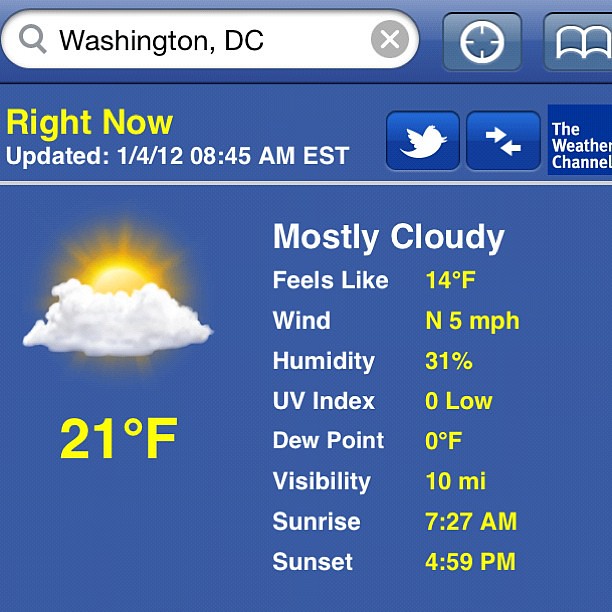This image is a detailed screenshot from a weather forecast displayed on a smartphone. The background is blue, with white and yellow text providing the weather details. At the top, there is a search bar with the text "Washington, D.C." and a magnifying glass symbol indicating it's a search field. To the right of the search bar, there are several icons: a gray circle with an "X," a white circle with four lines extending from the center, and a square outline with a book icon.

Below the search bar, a yellow label reads "Right Now," and in white text, it says "Updated 1-4-12, 8:45 a.m. Eastern Time." Next to this, there are three sharing options: a Twitter logo, a double-arrow symbol, and an emblem for The Weather Channel. The main part of the image, taking up the lower two-thirds, shows a graphic of the sun rising above clouds beside a yellow "21°F" and white "Mostly Cloudy."

Below the main weather image, details are listed in two columns: white on the left and yellow on the right. It states "Feels Like 14°F," "Wind: North, 5 mph," "Humidity: 31%," "UV Index: 0 (Low)," "Dew Point: 0°F," "Visibility: 10 miles," "Sunrise: 7:27 a.m.," and "Sunset: 4:59 p.m."